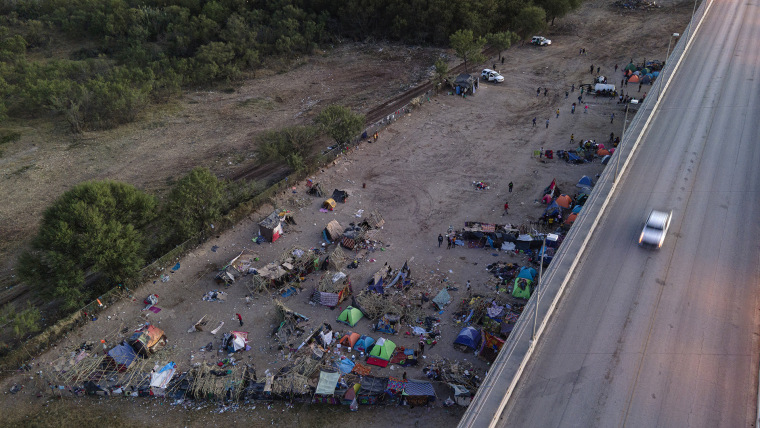This color photograph, taken from a drone, captures an area adjacent to a large highway on the right side of the image, where a single white car is driving towards the viewer. Dominating the middle section is a makeshift homeless campground, with various colored tents – including blue, green, and red – scattered across a dirt terrain strewn with trash. Several people can be seen walking around, some in small groups, while a couple of cars are parked nearby. Beyond the campground, close to the right edge of the image, runs a railroad track, bordered by more dirt and leading into a forested area. The entire scene is bathed in daylight, lending clarity to the chaotic yet colorful spread of tents and vegetation.